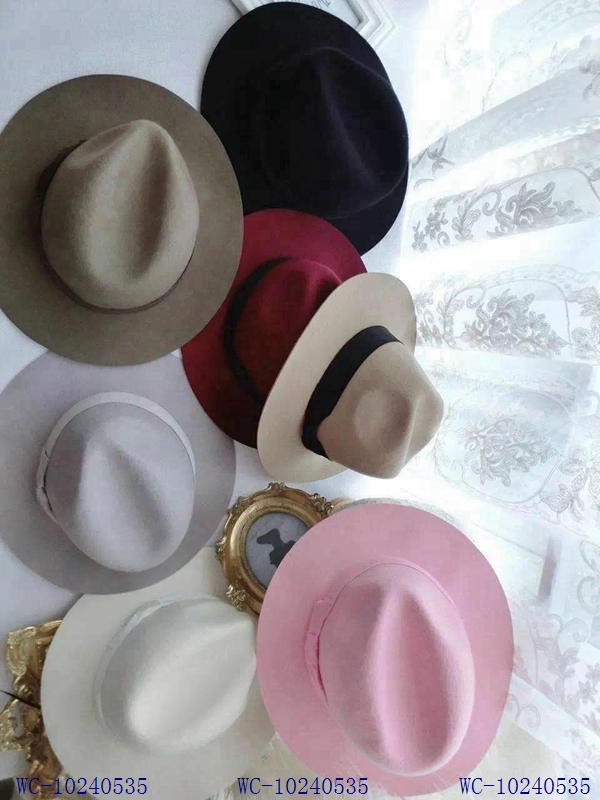The photograph, most likely taken in a living room or store, shows an overhead view of seven different colored hats, arranged in front of a lacy white curtain with a floral embroidery pattern filtering sunlight through closed windows. The curtain suggests a domestic or retail setting, enhanced by the ornate frame of a photograph featuring a black silhouette placed under the pink hat. The hats, which resemble fedoras or wide-brimmed southern-style hats, come in black, red, cream, white, gray, pink, and brown. The image is marked by a repeating watermark, "WC-10240535," at the bottom, possibly indicating a product page for second-hand goods. The overall presentation hints at the hats being organized for sale or display.